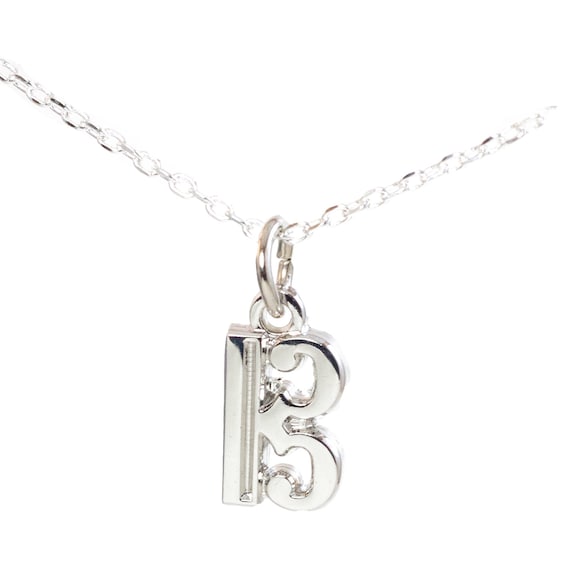A clear and detailed product image showcases a silver chain necklace against a white background, emphasizing its elegant design. The chain runs through a highly stylized amulet, which appears to depict either the number '13' or the letter 'B' in an artistic font. The amulet features an intricate looping structure, with one rectangle anchoring the design and additional loops extending both upward and downward from the center. The entire piece, including the chain and the amulet, gleams with a polished silver finish, likely sterling silver or sterling silver plated. The amulet is attached with a practical clasp mechanism, allowing for easy removal. The close-up nature of the image draws attention to the fine craftsmanship and intricate details of the jewellery piece.